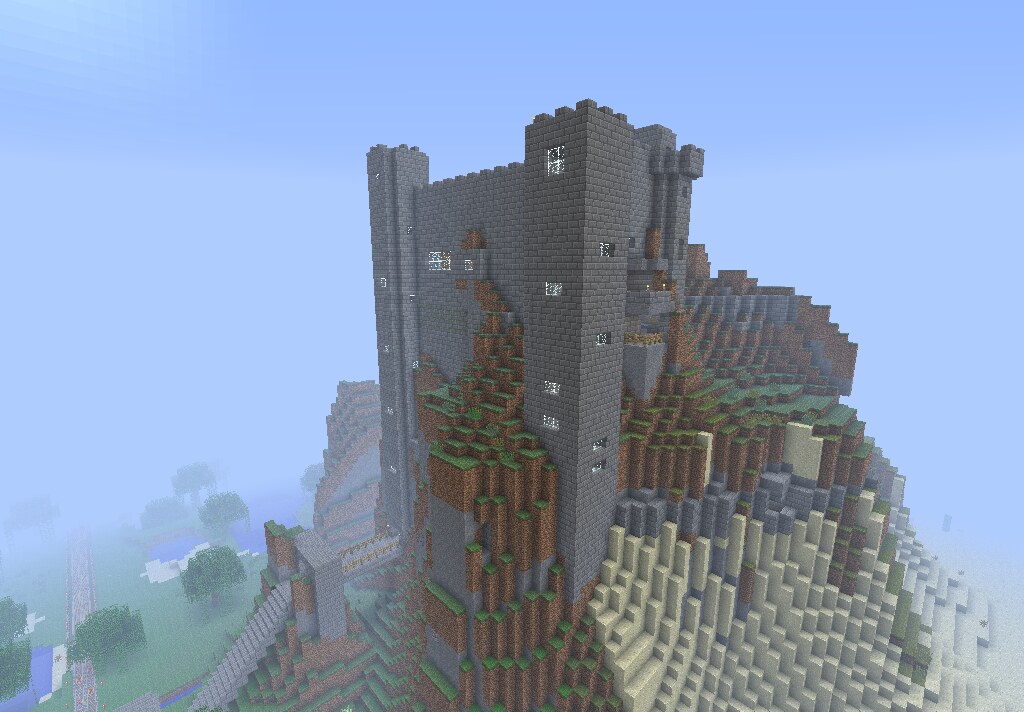The image is a horizontally oriented screenshot from a pixelated video game, likely Minecraft, depicting a large, multi-layered castle-like structure made predominantly of gray bricks. The imposing construction, which resembles both a tower and a castle, features random windows and is interspersed with patches of brown soil and green grass, giving it a partially demolished or under-construction appearance. To the left of the structure, the landscape includes a variety of natural elements: a ground covered with green trees that resemble tubes capped with grass, bodies of water, and a road leading up a grand staircase made of white, marble-like steps. The scene is set against a sky that shifts from darker blue at the top to lighter blue nearer the horizon, enhancing the detailed and vibrant colors of green, blue, brown, and white present throughout the image.